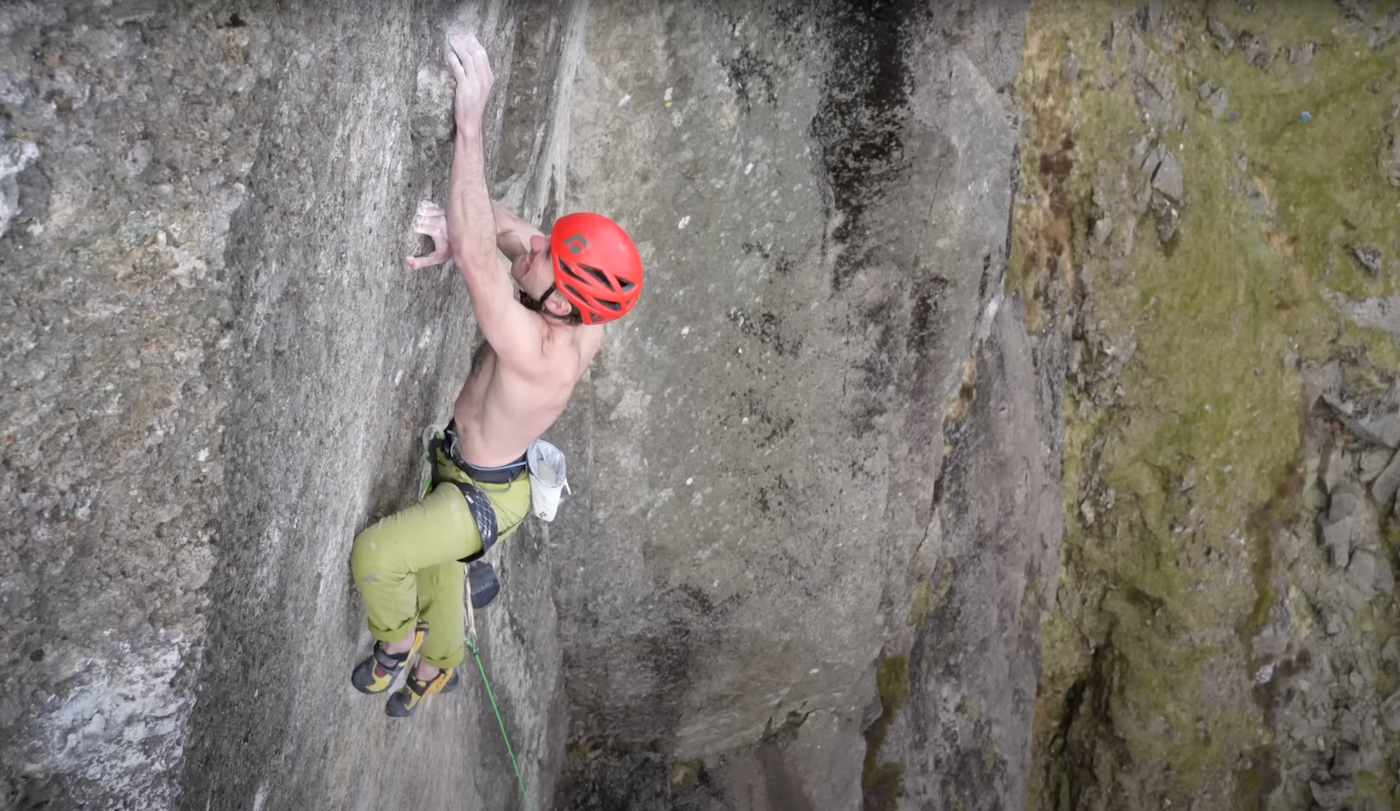The image depicts a young, shirtless man intensely climbing a nearly vertical, dark gray rock face. He's secured with safety gear, seen through black straps around his waist and upper legs, and has a red helmet for protection. The climber dons green pants and black and yellow specialized climbing shoes, and he's gripping tiny ledges with chalk-covered hands, making it hard to see what his feet are touching. Some additional equipment is clipped to his belt. The photo appears to be taken during the daytime, possibly by a drone or someone positioned above him, capturing his concentrated expression as he scales the daunting cliffside.